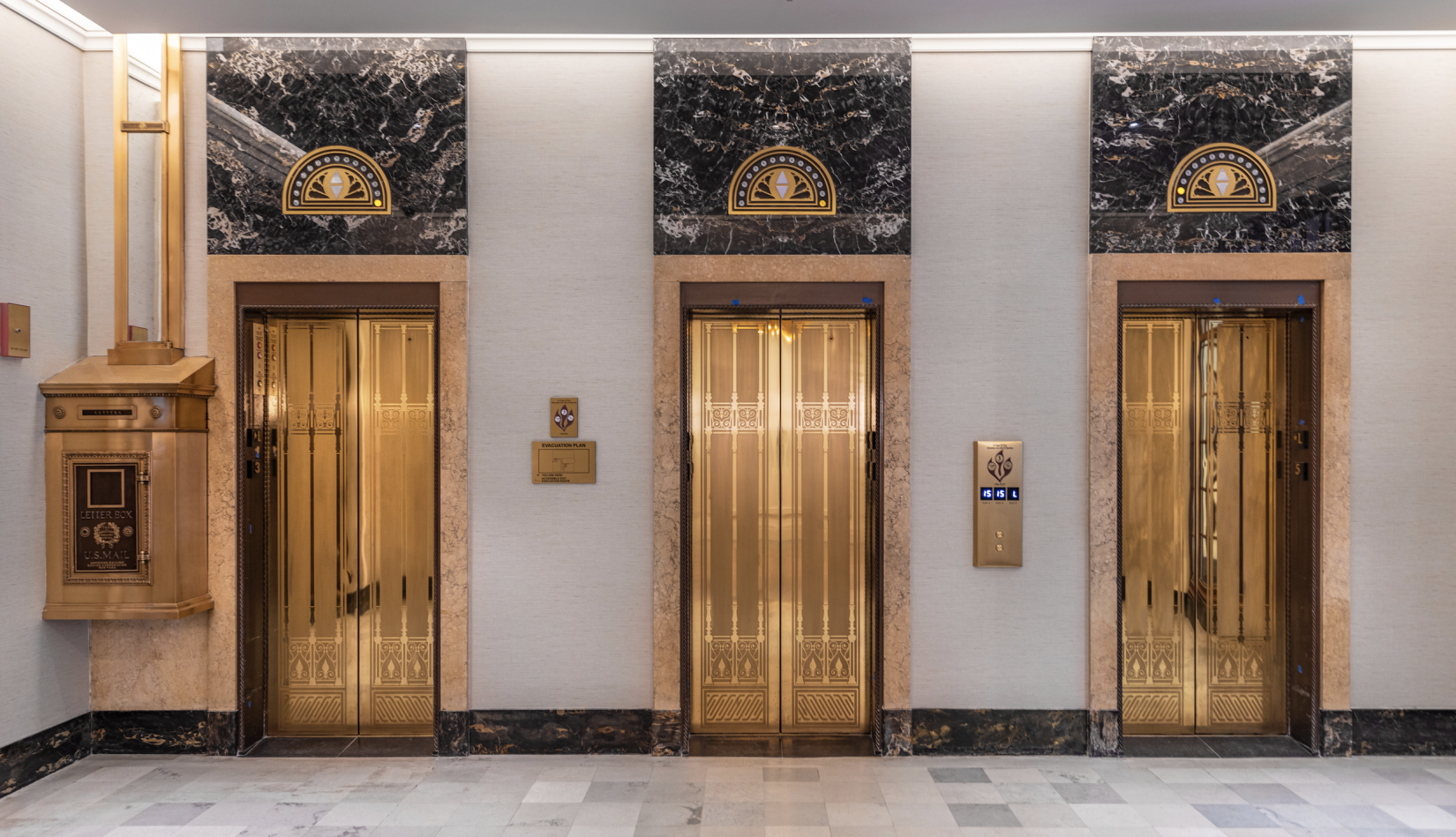The image depicts an elegant hotel lobby featuring three sophisticated elevators with a distinct steampunk flair. Each elevator sports gleaming golden doors and is framed by a black marbled arch, which houses a floor indicator displaying the current position of the elevator. The lobby walls are pristine white, adorned with various gold fixtures, including the elevator call buttons placed between the elevators and a notable large machine on the left side, crafted from gold or copper, adding to the steampunk aesthetic. The floor is tiled with various shades of white, arranged in a clean and orderly manner, complementing the luxurious ambiance of the space.